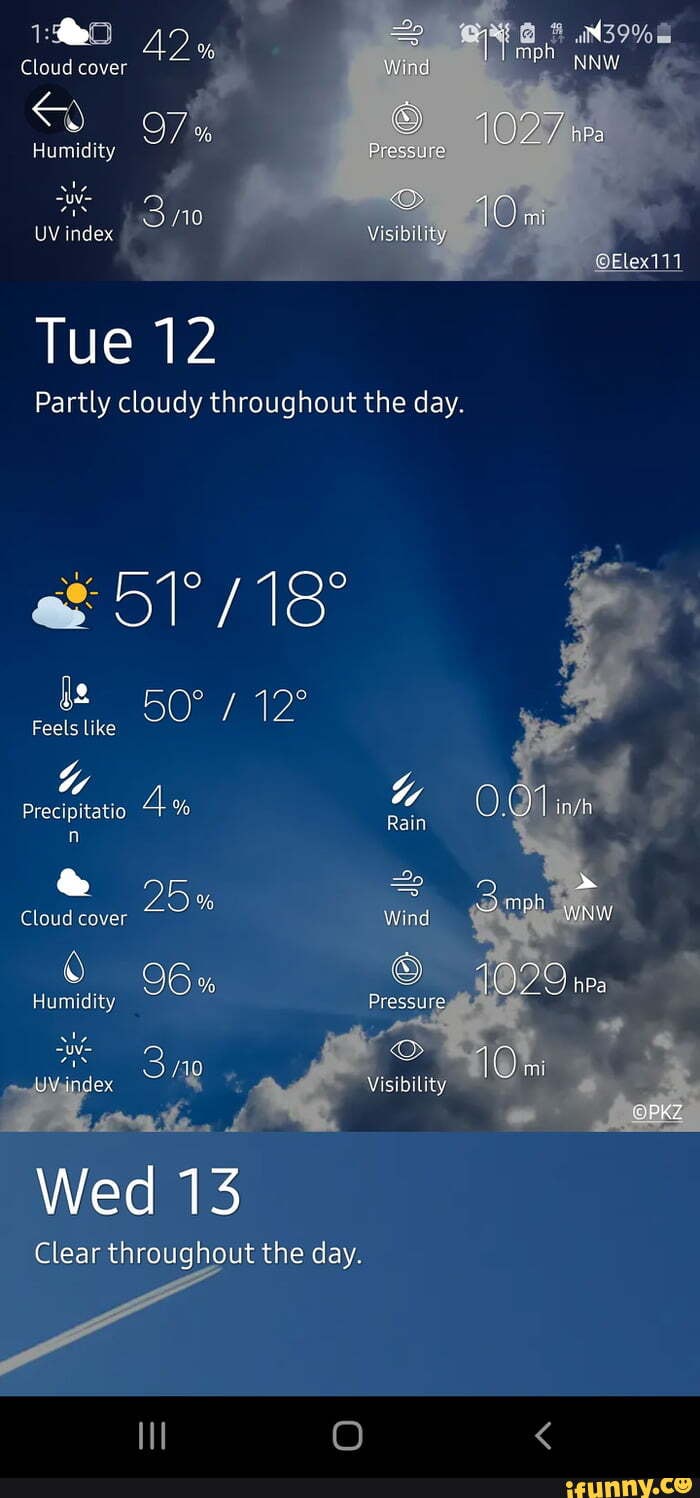The image depicts a mobile weather application on a smartphone. At the top of the screen, the status bar includes the current time on the left and right corners, as well as essential icons: an alarm clock, a silent mode indicator, and a battery icon showing a 39% charge. It also indicates signal strength and that location services are enabled. 

The main portion of the app provides detailed weather information. It displays a partially clouded sky with an icon representing clouds and the sun peeking through, suggesting 42% cloud cover. Key weather statistics like wind speed, barometric pressure, visibility, and UV index are prominently featured. 

Just below these metrics, the app shows the current date and weather summary, noting that it is Tuesday the 12th and partly cloudy throughout the day. The forecast also indicates a high of 51°F and a low of 18°F, with the temperature feeling like 50°F during the day and 12°F at night.

Further down, additional details such as precipitation levels, cloud cover, and humidity are listed along with a reiteration of the UV index. The left and right sides of this section cover rain probability, wind speed, pressure, and visibility in a descriptive format. 

Finally, the bottom segment of the app offers a brief outlook for the following day, stating that Wednesday the 13th will be clear throughout the day.